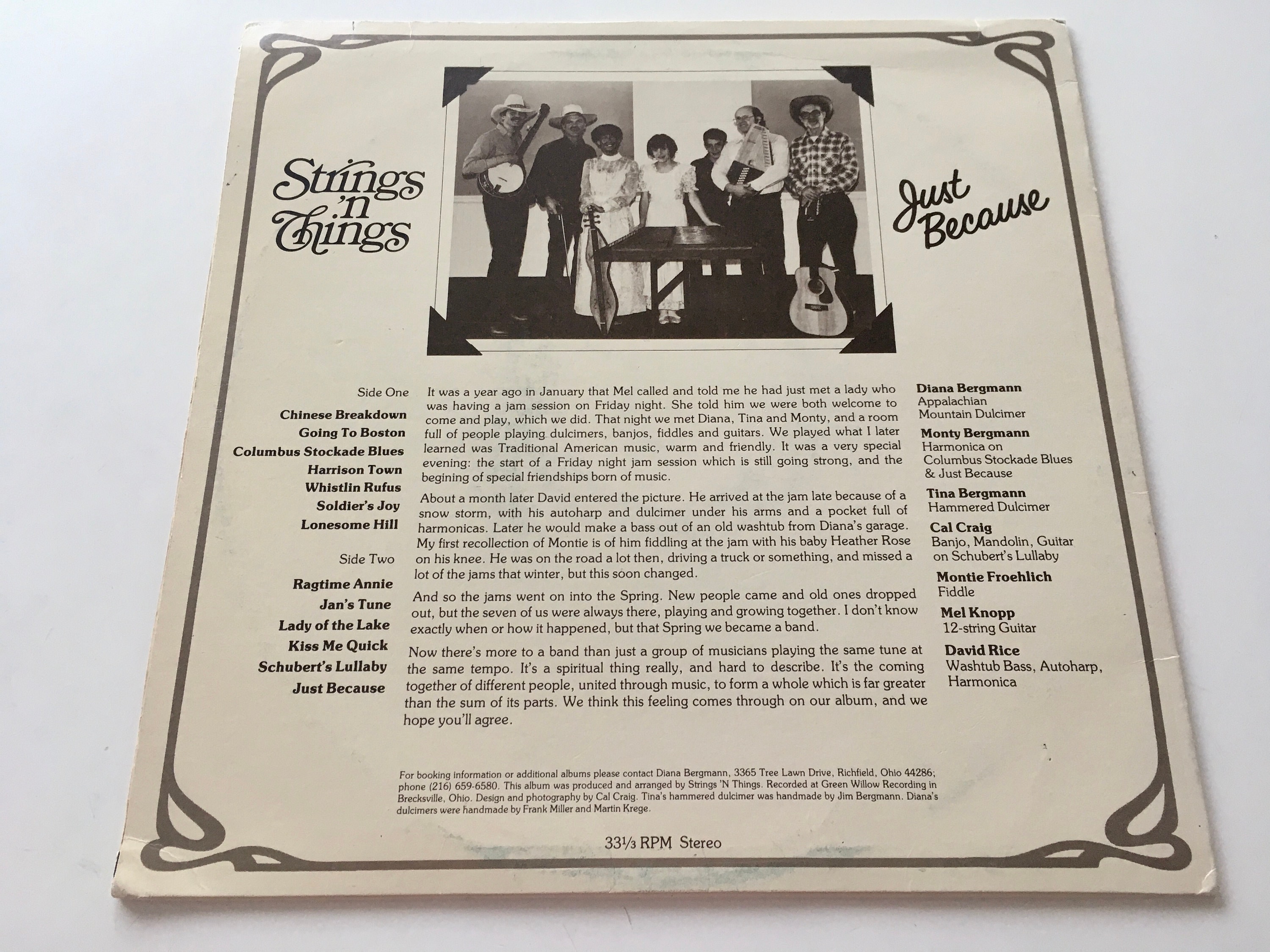The image is the back cover of a 33 1/3 RPM stereo vinyl record for the album "Just Because" by the band "Strings and Things." The cover is predominantly black and white, encased in a dark border. At the very top, there is a photograph of the band members—six in total, including men and women—each holding their instruments, such as guitars, banjos, and potentially a violin. Notably, there are two men in cowboy hats and a person in a plaid shirt.

On the left side of the cover, the title "Strings and Things" and the album name "Just Because" are prominently featured. Below, the track listings are provided: 

**Side One:**
1. Chinese Breakdown
2. Going to Boston
3. Columbus Stockade Blues
4. Harrison Town
5. Whistlin' Rufus
6. Soldier's Joy
7. Lonesome Hill

**Side Two:**
1. Ragtime Annie
2. Jan's Tune
3. Lady of the Lake
4. Kiss Me Quick
5. Schubert's Lullaby
6. Just Because

In the center of the cover, an extensive narrative details the band's backstory, highlighting their formation and experiences. This anecdote tells of how the band members met during a jam session and grew into a cohesive band, emphasizing their special bond and shared passion for traditional American music.

On the right, the individual credits for band members are listed:
- Diana Bergman
- Monty Bergman
- Tina Bergman
- Cal Craig
- Monty Froelich
- Mel Knopp
- David Rice

The cover also mentions technical production details and the personal stories of each member, further enriching the context of the album's creation and the band's journey.